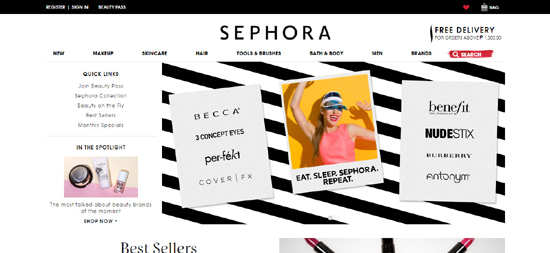The image features an online storefront for Sephora. The name "Sephora" is prominently displayed in the center of the page in black text. At the top of the page, there is a black background header with various elements. On the top-left corner, there's a "Register" and "Sign-In" option, along with "Beauty Pass." On the top-right corner, there is a red heart icon and a black cart icon. 

Centered below the main "Sephora" logo, there are several navigation tabs that include: "New," "Makeup," "Skincare," "Health," "Pools and Brushes," "Health and Body Bath." Additionally, a red search button is located on the top-right.

Above these tabs, a promotional banner states "Fleet delivery for orders above 300." 

The middle section of the page features a black and white background adorned with several brand stickers on the left and right sides. 

- Left side stickers: "Becca," "J-concept," "Eye Perfect," and "Cover FX."
- Center image: A man wearing an orange vest against a yellow background with the text "Eat, Sleep, Sephora, Repeat."
- Right side stickers: "Benefit," "Nude Sticks," "Burberry," and "Antonym."

Additionally, there are quick links like "Join Beauty Pass," "Beauty on the Fly," "Bestsellers," and "Monthly Specials."

At the bottom of the page, there is a section titled "In the Spotlight," showcasing detailed images of makeup products. Below this, there is a "Bestsellers" section. In the bottom-right, there are rouge icons in black and red.

This detailed description encapsulates the visual layout and the navigational and promotional elements of the Sephora online store’s webpage.